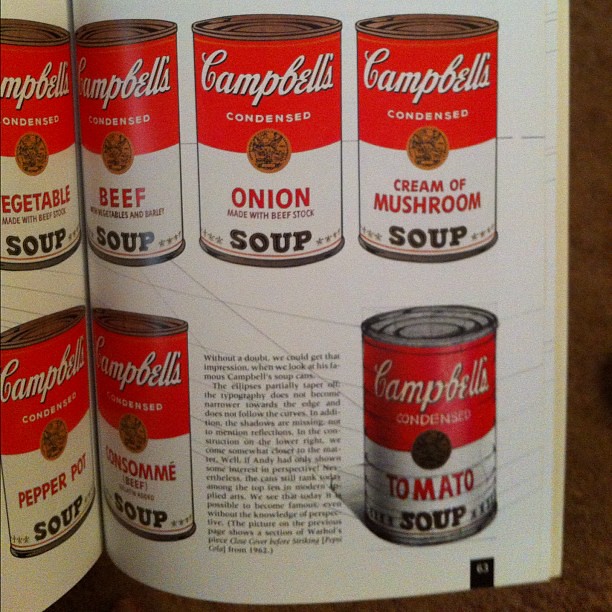The image captures a first-person perspective photograph of an open magazine, positioned against what looks like a wooden tabletop. Both pages of the magazine are displayed, revealing a vintage advertisement for Campbell's soup. The advertisement features multiple cans of various Campbell's soups, including Condensed Vegetable Soup, Beef Soup, Onion Soup, Cream of Mushroom Soup, Pepper Pot Soup, Consommé Soup, and Tomato Soup. The cans are meticulously arranged, with five on the right page: three on the top half—Beef, Onion, and Cream of Mushroom—followed by Consommé and Tomato on the bottom half.

A descriptive paragraph is nestled between the cans on the right page, presenting an analysis of the iconic Campbell's soup cans, associated with Andy Warhol's artistry. The text critiques the typographic and visual aspects of Warhol's work, emphasizing its modern influence despite a lack of traditional perspective. Additionally, the magazine features a small black box in the bottom right corner of the right page, indicating it is page 63, and shows mild signs of aging with slightly yellowed edges.

The magazine's appearance and the design of the soup cans give it an old-fashioned charm. In the background on the right edge of the image, a small section of brown carpet is visible, adding another layer of context to the setting.